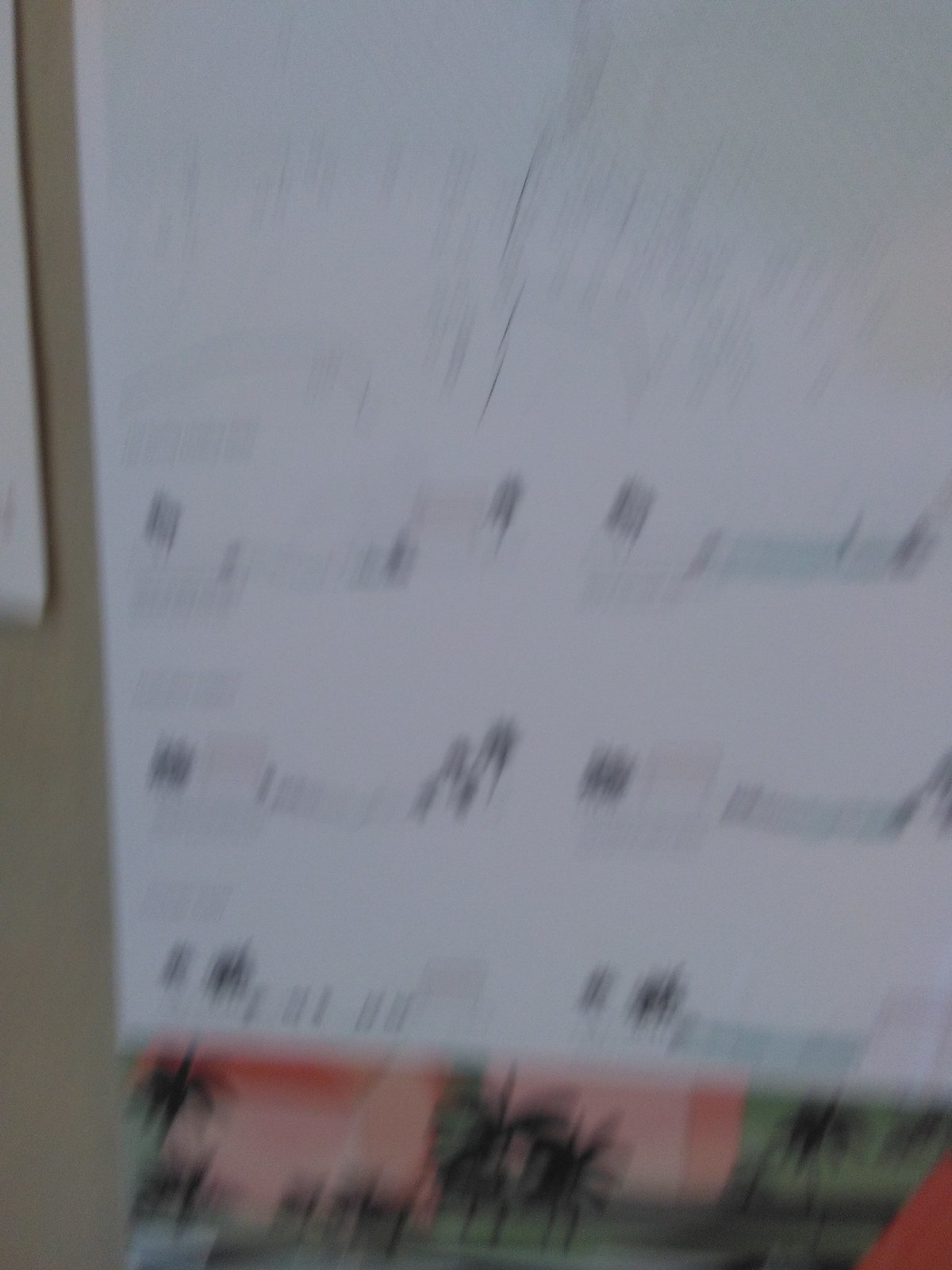This blurry photograph appears to capture a giant wall-mounted poster segmented into two primary sections: an upper half dominated by a large, indiscernible diagram and a lower half divided into six distinct sections. Each section prominently features graphical designs, though their specific details remain vague due to the image's poor clarity. The bottom of the poster showcases a banner adorned with black palm trees set against alternating pink and green backgrounds, evoking a tropical theme. The arrangement might suggest themes or days typically found in a calendar, especially as numbers seem to evenly space across part of the image, resembling date placements. The overall presentation and context hint at an educational or corporate environment, rather than a personal one, with potential mathematical functions involved, albeit unreadable. The entire poster is affixed to a dark cream-colored wall, adding to the impression that this is a functional decor piece for informative or organizational purposes.